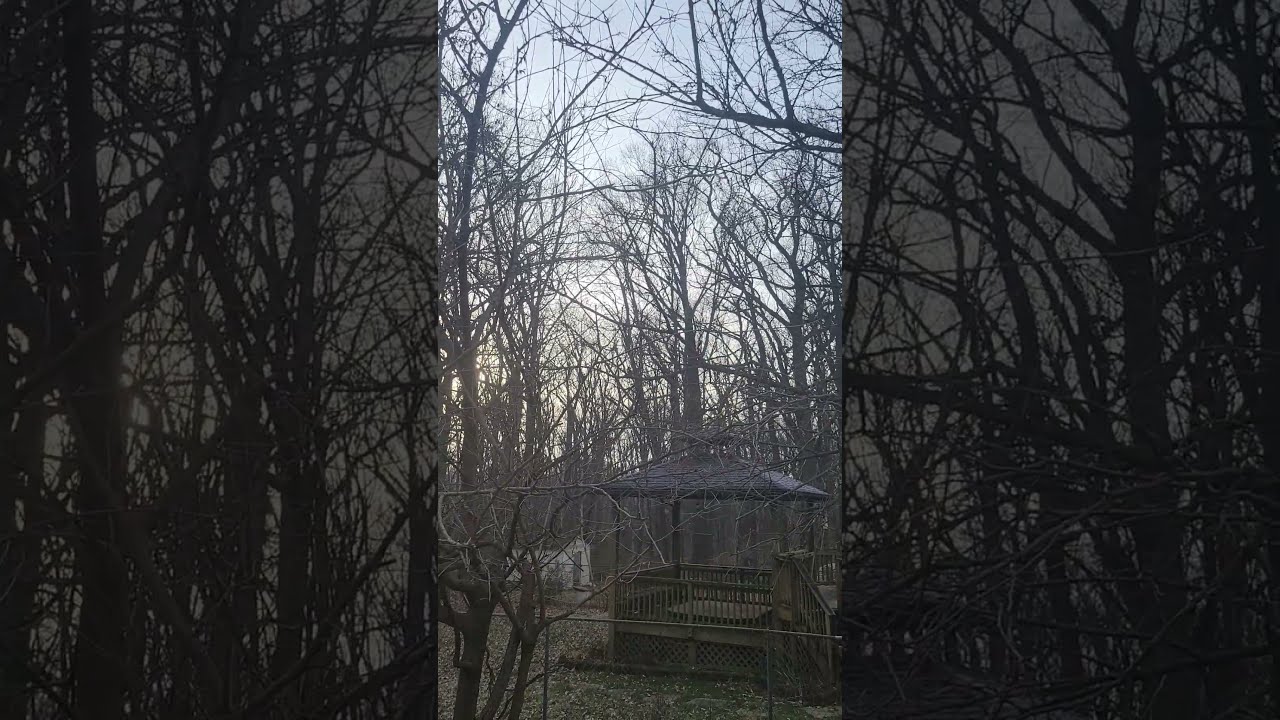The image captures a serene outdoor scene, likely taken during the winter season given the absence of leaves on the trees. Dominating the lower portion of the image, we see a well-defined ground covered with a mix of grass and fallen brown leaves. A chain-link fence runs along the bottom of the frame, just beyond which lies a hexagonal gazebo situated in the bottom right corner. This wooden gazebo, elevated slightly above the ground with lattice work underneath and a low railing around it, is accessed by steps with visible wood railing. In the lower left foreground, there's a seemingly lifeless bush without any leaves. Beyond the gazebo, the background is filled with numerous leafless trees extending into a grayish-blue sky, which takes up most of the upper part of the image. Toward the far left, a small, light gray building can be seen in the distance. The overall color scheme consists of blue, gray, white, black, tan, and green. The image appears to be a screenshot taken from a mobile device and includes a dark, partially blacked-out border, indicating some level of image manipulation or enhancement. The setting conveys a tranquil, mid-day atmosphere within a deciduous forest area.